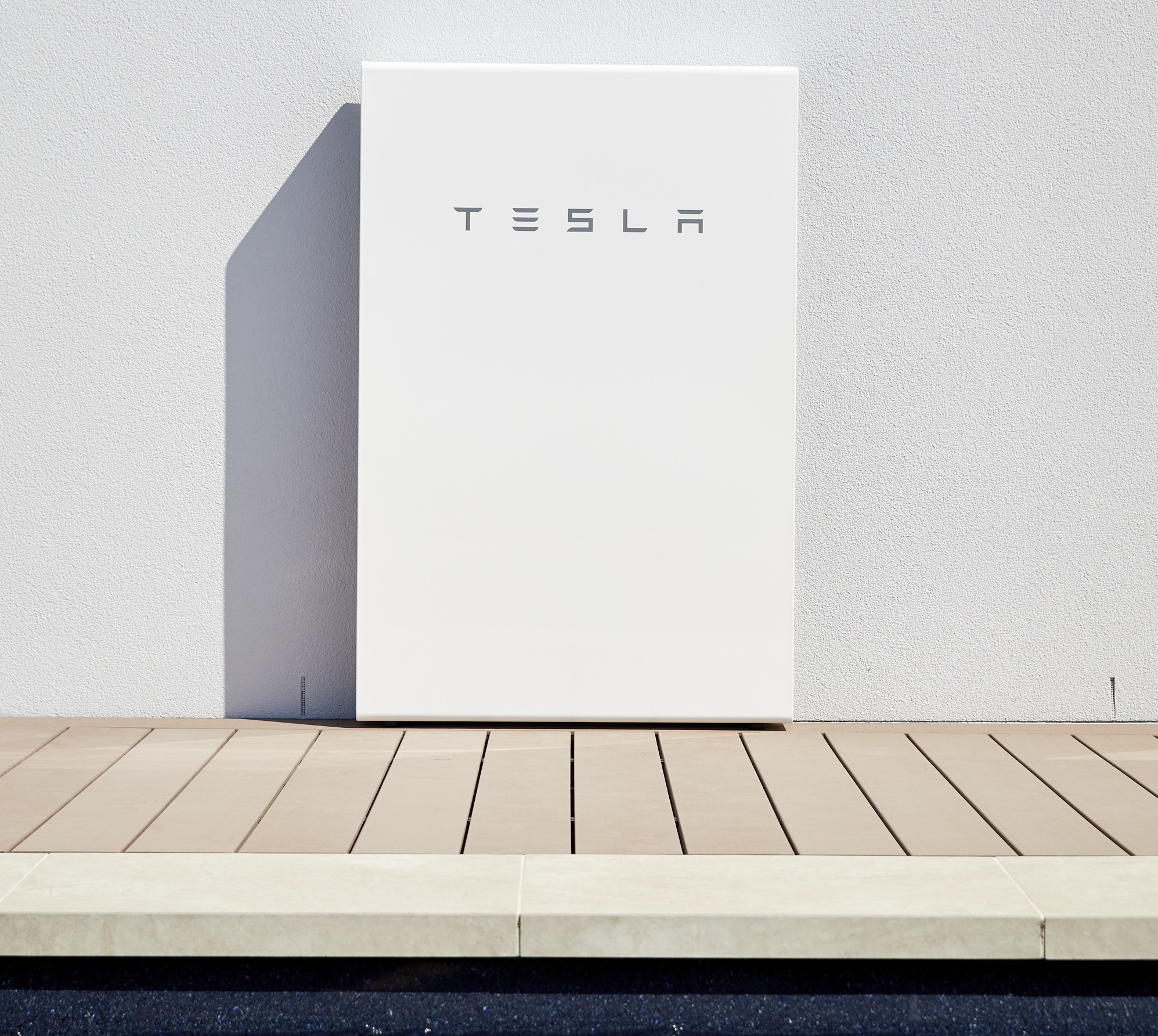This photo showcases a Tesla home battery, presented as a substantial white box adorned with the sleek grey Tesla logo on its front. The unit is securely mounted to the grey, concrete-painted wall of a house. Beneath the battery, just a couple of inches away, lies a narrow brown wooden sidewalk fashioned from horizontally arranged boards, each spaced roughly two inches apart. Flanking this wooden walkway are thin concrete blocks, meticulously aligned with white grout visible between each one. The bottom edge of the photo reveals a layer of black, glass-like gravel, which neatly borders the walkway, enhancing the overall aesthetic of the setup.